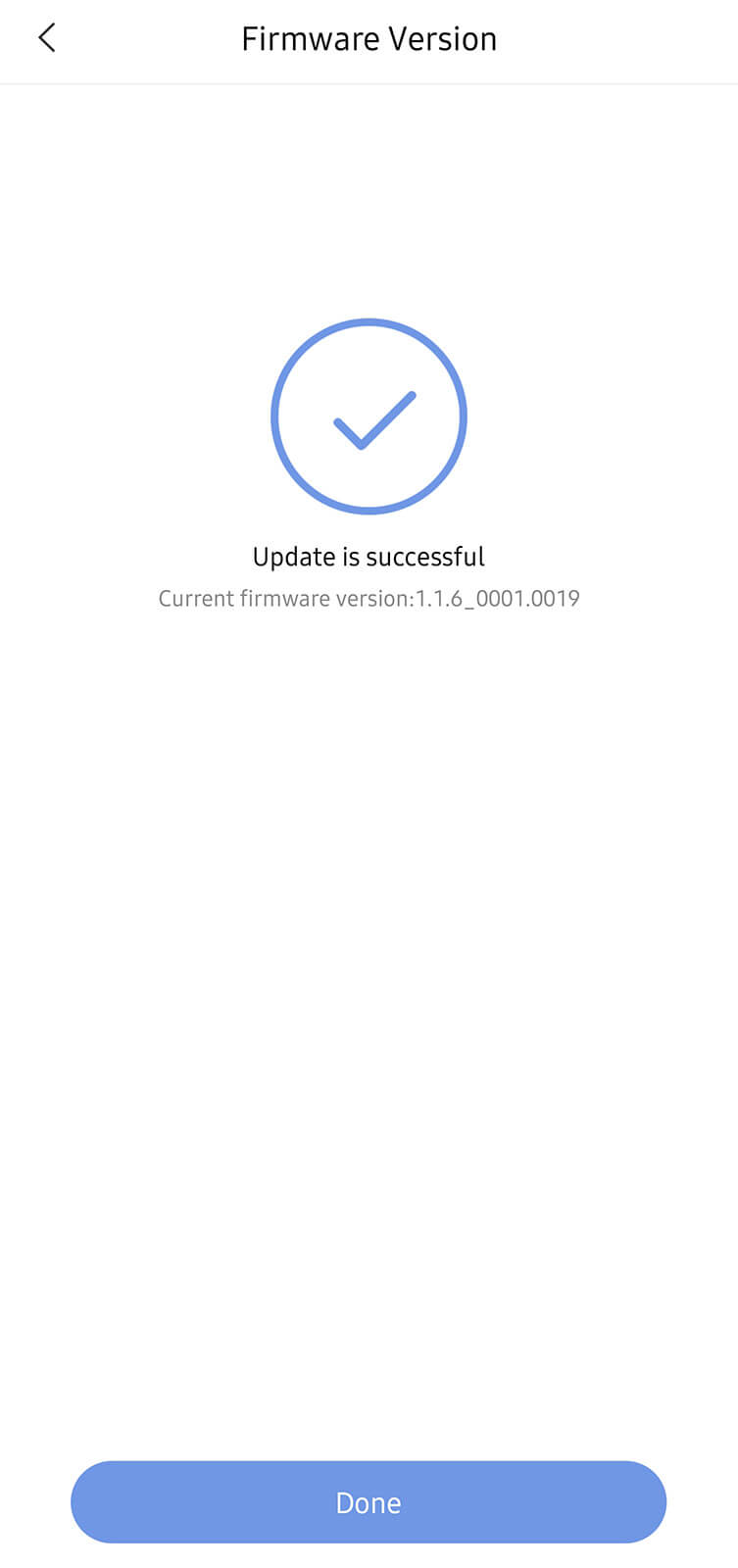The image features a screenshot with a standard white background, resembling a phone interface. Positioned at the top-left corner is a black arrow icon, resembling a sideways "V" pointing left. Adjacent to this icon, in black text, are the words "Firmware Version."

Just below this header, a thin gray line spans horizontally, demarcating the header from the main body of the screenshot. The main section of the page is solid white and centrally features a blue circle encompassing a blue checkmark.

Beneath the blue circle, bold black text reads "Update is successful." Following this, in regular gray text, is the statement, "Current firmware version: 1.16_0001.0019."

At the bottom of the screen, a rounded blue button extends the full width of the image. Centered within this button, in white text, is the word "Done."